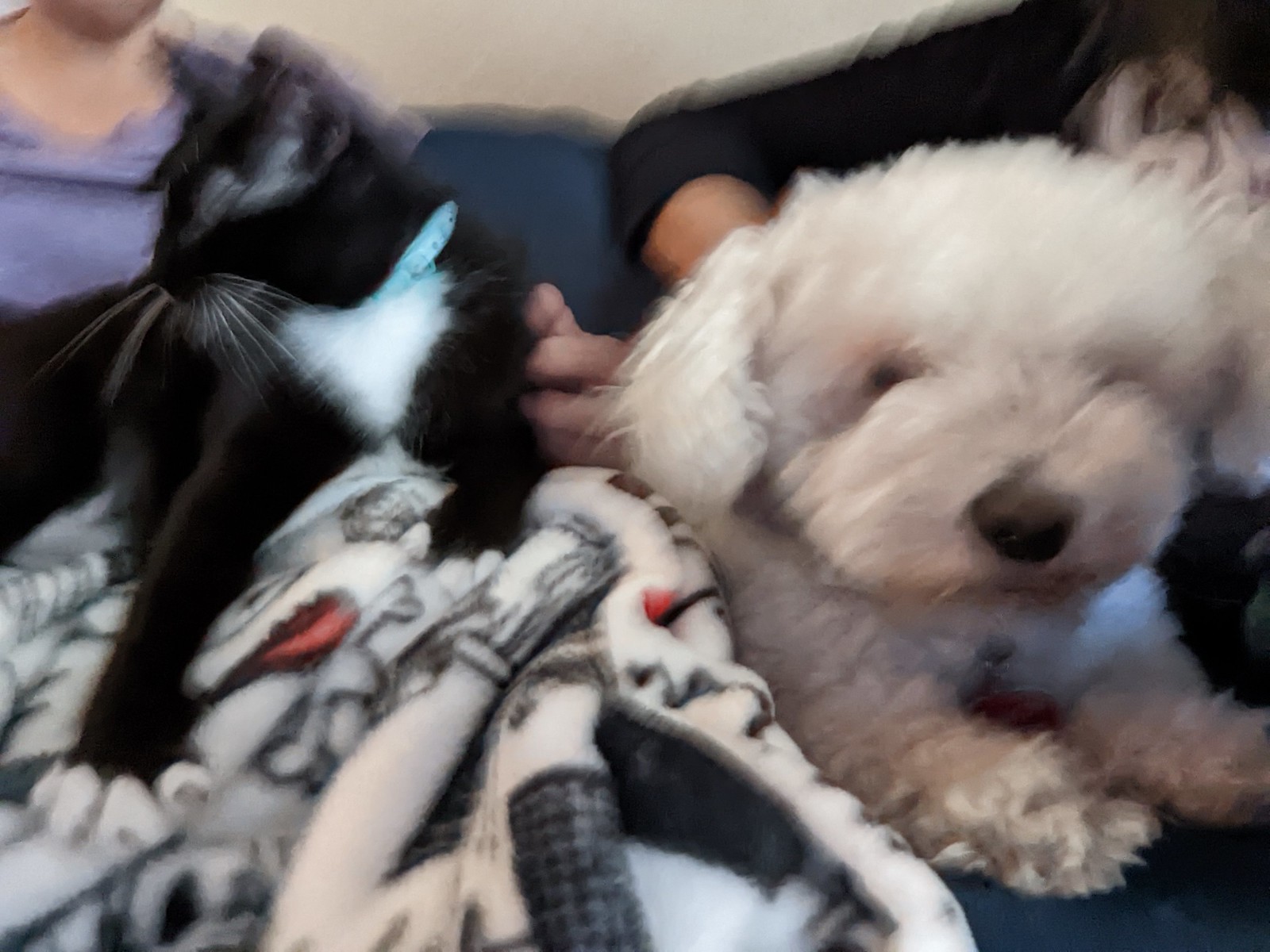In this slightly blurry image, a cozy scene unfolds on a couch. A black and white cat with a light blue collar sits comfortably, seemingly perched on someone's lap. Beside the cat, a small dog, likely a Bichon Frise with its characteristic curly white fur, sits contentedly. The dog has a typical black nose and bears the familiar, endearing look of lap dogs. 

Two individuals flank the animals, their faces out of view. On one side, the person wearing a long-sleeve black hoodie with a visible logo has their arm casually draped over the back of the couch. On the other side, a person in a light purple short-sleeve t-shirt sits close, completing this intimate family tableau. Despite the blurred focus, the image captures the warmth and companionship shared among the group.